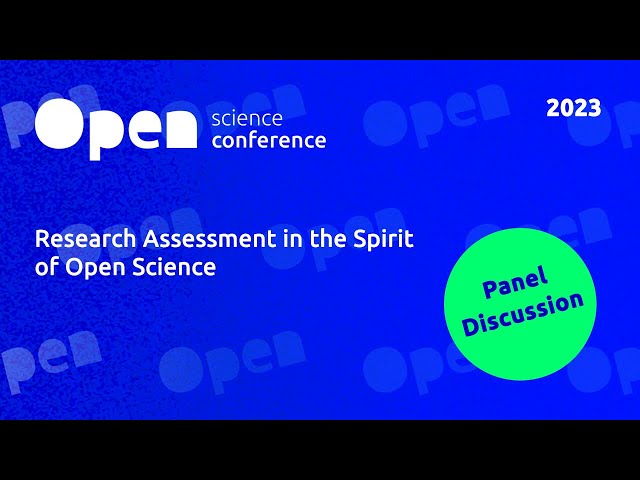The image is a screen capture of an introductory slide for the Open Science Conference 2023. The slide prominently features the title "Open Science Conference 2023" positioned on the top left, with the subtitle "Research Assessment in the Spirit of Open Science" underneath. There is a notable "Panel Discussion" text on a green circular background towards the bottom right. The slide design includes band-like black and white borders at the top and bottom, reminiscent of a movie frame, with the rest of the background being blue. Repeated instances of the word "open" are subtly visible throughout this blue background. The design is minimal, lacking specific details about the date beyond the year 2023 and appears to serve as an online ad or informational slide for the conference. The overall aesthetic and layout clearly point to this being an initial or introductory slide within a larger presentation.